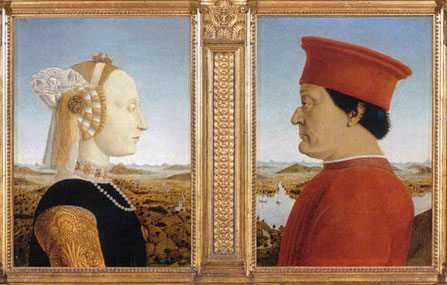This image is a detailed painting split into two sections by an ornate golden border, creating the appearance of two separate yet connected portraits. Both sides are framed together in a lavish golden frame. 

On the left side, the painting depicts a woman with blonde hair styled into a bun, adorned with a white flower-like decoration. She is wearing a black dress with golden sleeves and two necklaces - one gold and one pearl. She has a fair complexion and is facing sideways, her gaze fixed on the man in the adjacent portrait.

The right side features a man with black hair, wearing a red smock that resembles a robe and a large red hat, similar to a Fez. He has a slightly darker complexion compared to the woman and is also looking directly at her.

The shared background of the painting includes a dirt mountainy region with a serene lake, trees, and a blue sky, creating a cohesive and scenic backdrop for both figures. The intricate border separating the two portraits is about three or four times thicker than the rest of the frame, adding to the ornate nature of the artwork.